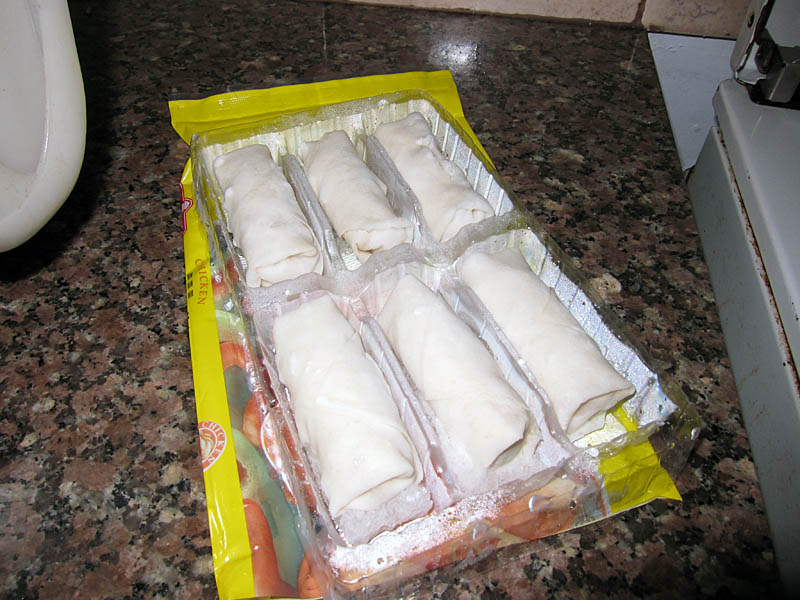This color photograph showcases a package of frozen chicken burritos. The image captures a plastic tray with six individual compartments, each holding a large, white, folded burrito. The tray itself sits atop a yellow plastic bag, which prominently displays the word "chicken," indicating the burrito filling. Positioned on a distinct granite countertop with notable pink and red hues, this kitchen setting possibly uses the microwave or stove to heat the frozen burritos, making them ready for consumption. The burritos, aligned in two rows of three, exhibit the characteristic folds and significant size that distinguish them from similar foods like spring rolls or chimichangas.